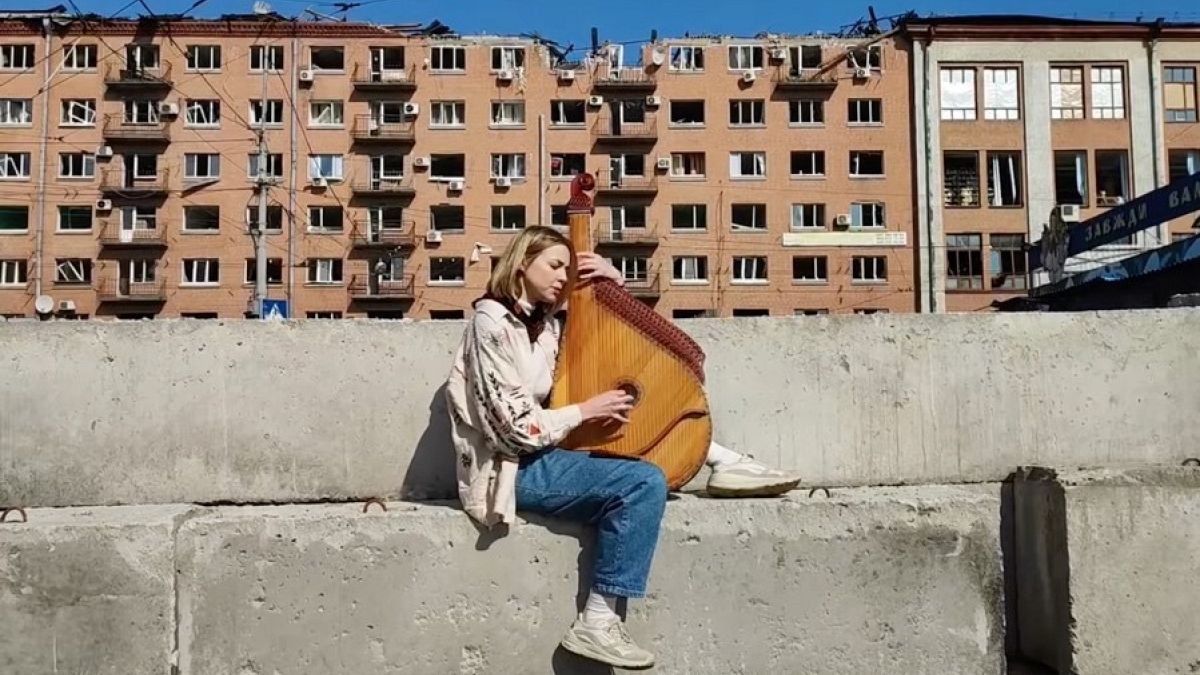In the colorful rooftop image, a young woman in her 20s, with shoulder-length blonde hair combed straight down, sits sideways on a concrete ledge made from large cement blocks. She wears a long-sleeved white jacket, blue jeans, and white sneakers. Her right leg dangles down the side of the wall while her left leg is propped up. She cradles a unique, traditional-looking instrument resembling a large dulcimer with a round, blond wooden body, numerous harp-like strings, and a guitar neck.

The backdrop features tall, slightly run-down, reddish-brick apartment buildings with some broken windows, enhancing an Eastern European vibe. On the right side, another building with a brownish-type roof and larger windows stands out. A blue crane with Cyrillic writing nearby hints at the location’s possible Greek or Russian influence.